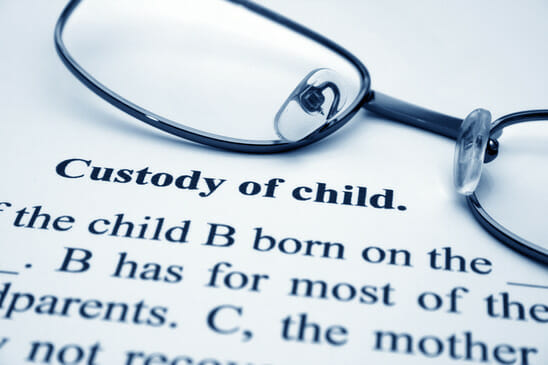This image is a tightly cropped black-and-white photograph of a legal document on pure white paper. Centered on the document, in bold typewriter-style black text, is the title "Custody of Child." Positioned over the document is a pair of prescription glasses with black frames and clear nose pads. The left lens is fully visible, while the right lens is only partially shown due to the zoomed-in nature of the photo. Beneath the title, fragmented lines of text read: "The child, B, born on the...," "B has for most of the...," "Parents... C, the mother...," indicating key details about the document but without complete sentences due to the cropped view.